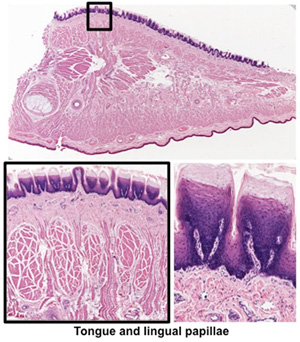The image is a detailed collection of three microscopy slides focusing on the anatomy of the tongue and lingual papillae. The top rectangular slide features a section of tongue tissue, rendered in a palette of muddy pinks, purples, and whites. This section contains a notable black box highlighting a specific area. The two bottom images, arranged as squares, are close-ups and appear to be scientific illustrations that explore this highlighted section further. 

The bottom left image zooms in on the intricate, tangled webs and structures akin to a side view of teeth, though they are not teeth. The detailed drawing shows a cross-section with purple and white areas, giving an impression of fine details within the tongue's tissues. The bottom right image offers another close-up, focusing on the purple divots and small lines denoted by the black square from the top image. Together, these illustrations exhibit the complexity of the tongue's inner structures, such as the lingual papillae, with detailed anatomical insights annotated and given precision.